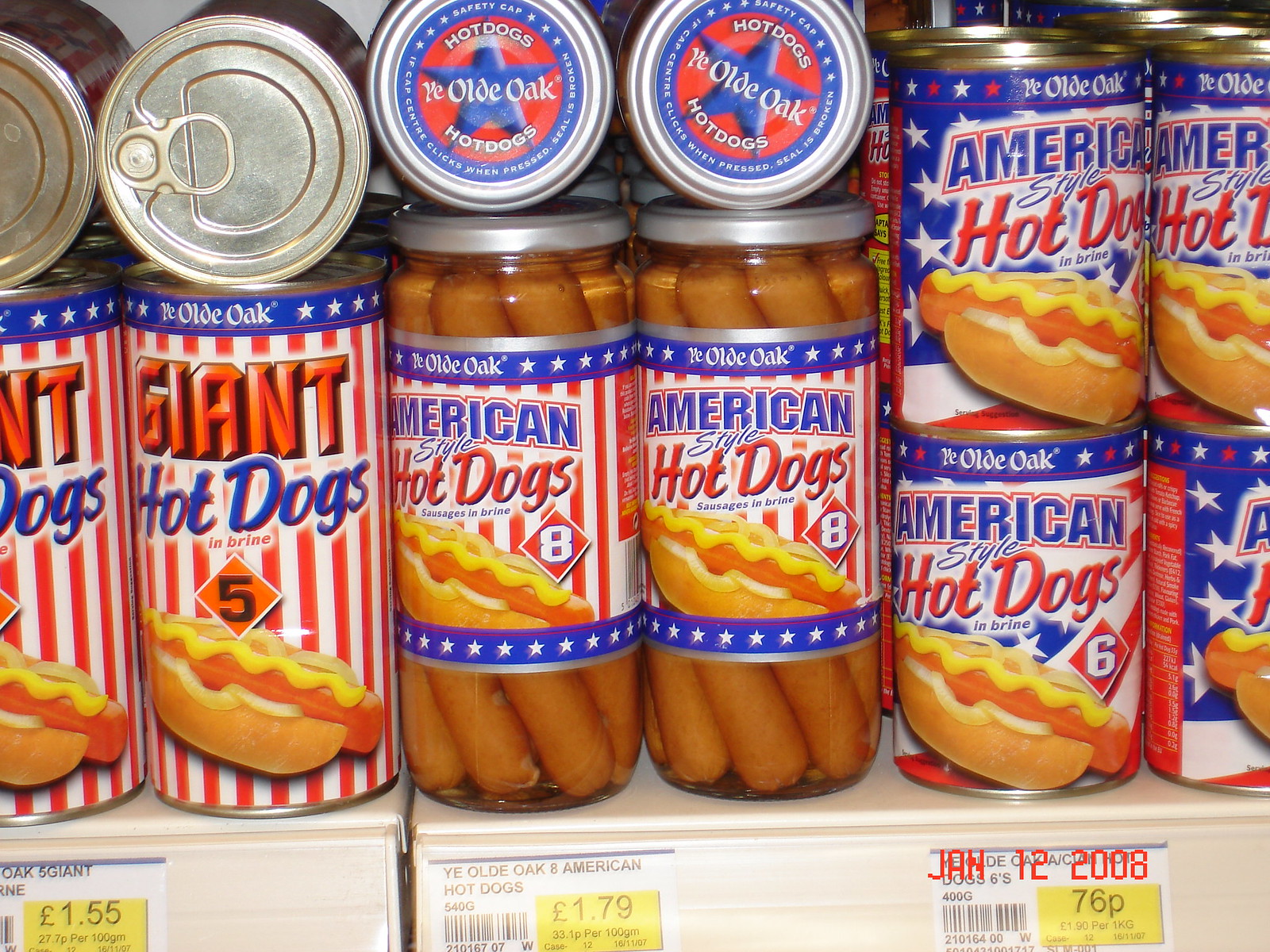The image captures an up-close view of a store shelf laden with various packaged hot dogs, indicated by the price cards denoting prices in British Pounds, suggesting the location is somewhere in the United Kingdom. The date stamped on the image reads January 12, 2008. 

To the left, there are tall tin cans of "Ye Olde Oak Giant Hot Dogs" prominently displayed. These cans feature a distinct red and white vertical-striped design with a blue border adorned with white stars at the top. The label displays "Ye Olde Oak" in the center with "Giant Hot Dogs" prominently written in large letters — "Giant" in bold red with a black border, and "Hot Dogs" in blue with a red border underneath. Below these, in smaller red letters, it states "In Brine." The can showcases an angled image of a hot dog on a bun accompanied by mustard and what appear to be onions, with an orange triangle and the number five in black at the center.

To the right of these cans, there are tall, round glass jars filled with hot dogs. These transparent jars allow a clear view of the hot dogs inside, capped with silver lids. They feature a similar red-striped label as the tin cans. At the top of the label, it reads "Ye Olde Oak" within a blue banner decorated with white stars. In the middle, it says "American Style Hot Dogs," with "American" in blue, "Style" in a small font, and "Hot Dogs" in large red letters. Towards the bottom right of the label, a red triangle with a white number eight and the familiar angled hot dog image is displayed.

Further right, a smaller tin can labeled "American Style Hot Dogs in Brine" is visible. This variant has an American flag design replacing the red and white stripes featured on other cans. It states "Six Hot Dogs" instead of five or eight, aligning with the uniformity of the product presentation, including the recurring bun-and-mustard hot dog image.